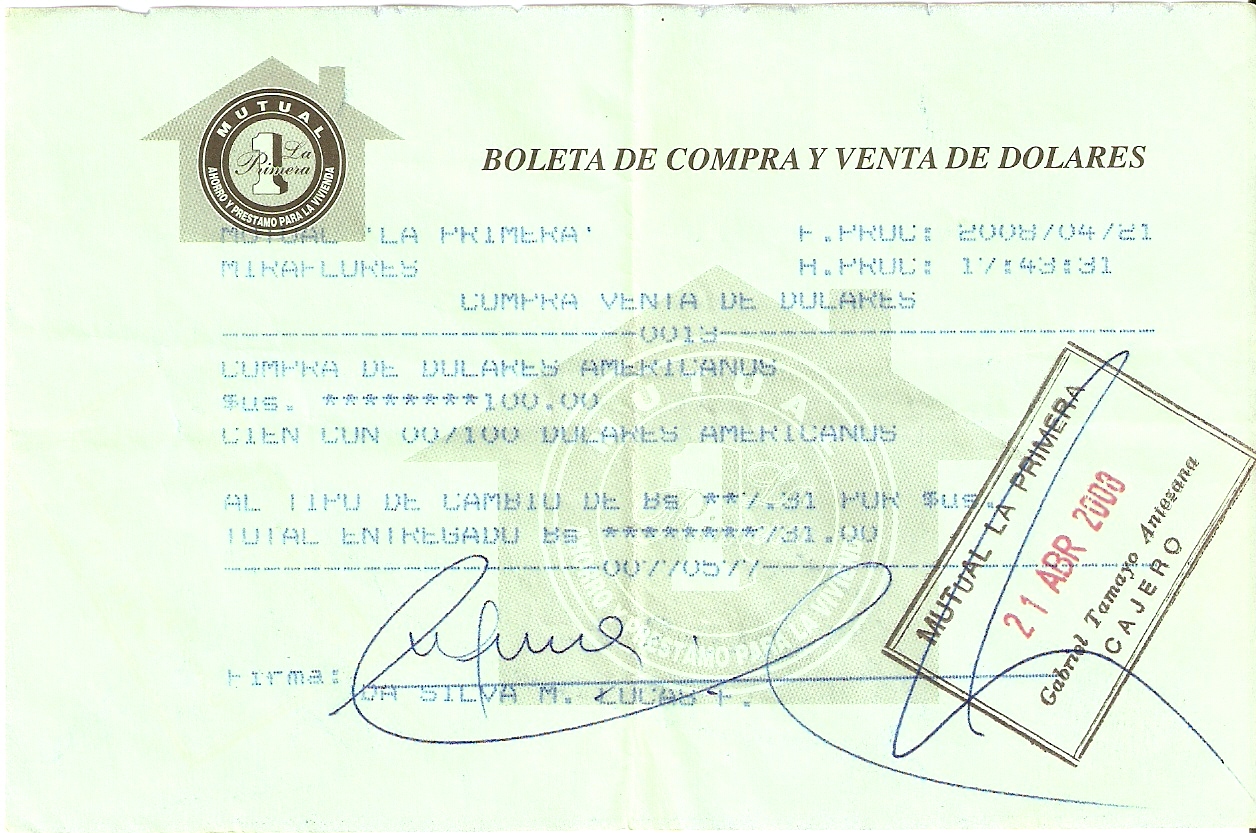The image features a note containing the following details: the words "boleta" (which can be spelled as "bolete" or "boleta"), "de compra y venta" (which translates to "of purchase and sale"), and "de dólares" (meaning "of dollars"). There is a photograph of a house with the word "Mutual" prominently displayed. Additionally, the note includes a stamp or seal that reads "Mutual Love Primera." The date on the stamp is "21 Abr 2003," indicating April 21, 2003. The note also contains the name "Gabriel Tamayo Antasena" followed by the word "cajero" (which translates to "cashier").